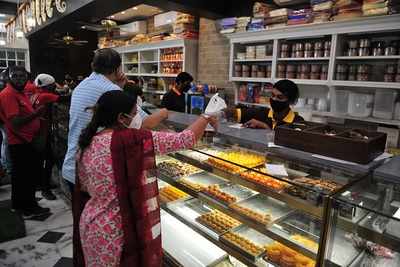The image depicts a bustling deli, possibly doubling as a bakery or sweet shop, with a glass display case showcasing various food items and desserts, predominantly orange, yellow, brown, and white. Many trays in the display case appear nearly empty, suggesting high customer turnover. At the counter, a woman in a red outfit and face mask appears to be purchasing sweets or other items from an employee. The employee, clad in a black polo shirt with a yellow collar and a black face mask, is busy assisting her. Another customer, a man in a light blue polo shirt with white stripes, stands beside her, seemingly awaiting service. Behind the employee, shelves laden with jars and other products line the back wall. Additional customers, including three men in red shirts, wait further down the counter. The colors prevalent in the image include yellow, orange, maroon, blue, black, red, and white, and the scene appears to be set around lunchtime.